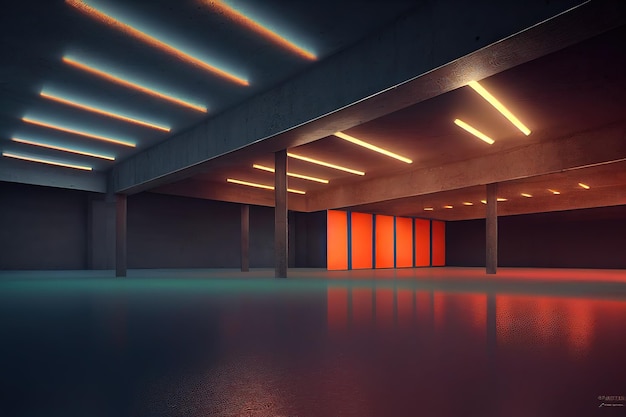The image depicts a vast, likely computer-generated space that could be part of a corporate or professional structure, resembling a parking garage or a commercial building's basement. The scene showcases gray floors and ceilings intersected by white beams of light, with additional gray beams extending from the ceiling to the floor. These elements create a modern, somewhat industrial atmosphere. A sizable section of the image features six interconnected orange walls with blue bars separating them, contributing to a vibrant contrast with the predominantly monochromatic setting. This area is distinctly illuminated, with the orange light reflecting off the floor, giving the surface a glossy, almost wet appearance. The overall color palette includes black, white, gray, blue, orange, red, and pink hues. Notably, the space is devoid of any human presence. In the bottom right-hand corner, there's a white text detail, though it is too small to decipher.